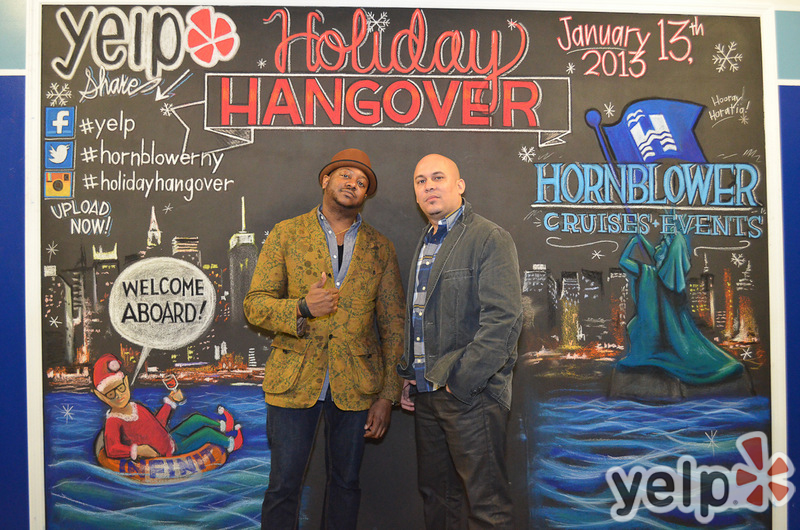In the image, two men are standing in front of a colorful, chalkboard-style advertisement for a Yelp-sponsored "Holiday Hangover" event, which took place on January 13, 2013. The backdrop features an artistically drawn New York City skyline with vibrant blues, reds, whites, and oranges. On the right side, there's text that reads "Hornblower Cruises and Events," and a whimsical depiction of the Statue of Liberty holding a flag while floating in the water with a Santa Claus character in an inner tube. Social media logos for Facebook, Twitter, and Instagram are also present. The man on the left, who appears to be African American, is dressed in a brown top hat with an elaborate beige, orange, and brown patterned suit jacket over a blue undershirt and jeans. The man to his left is bald, possibly Hispanic, wearing a gray jean jacket over a blue flannel shirt, with his hand in his pocket and dressed in black pants. They stand poised against the vivid, holiday-themed chalk drawing, which reads "Holiday Hangover" in large, festive red text.